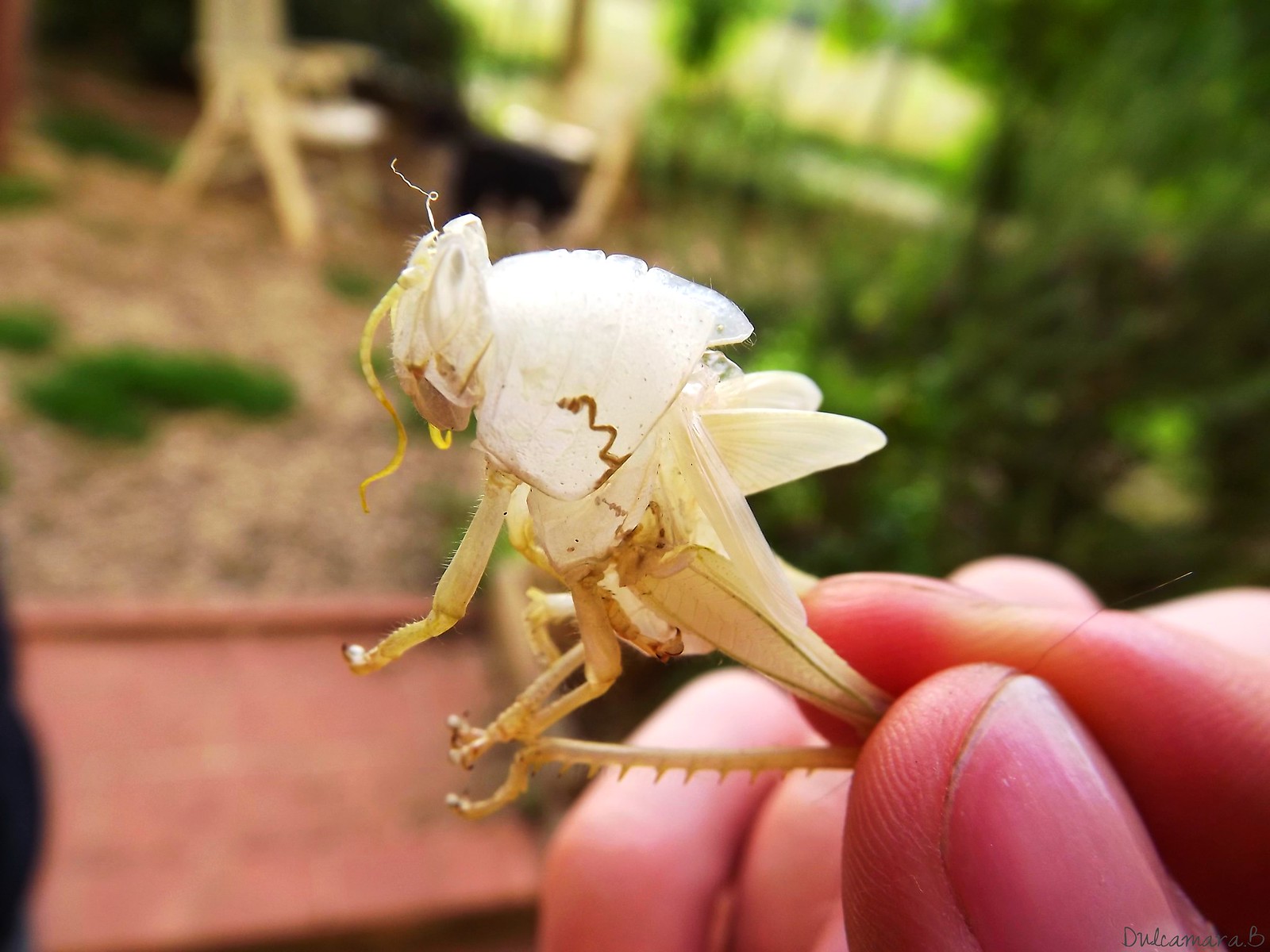In the photograph, we see a close-up of a person's hand with fairly tan, pinkish skin, holding a translucent cricket or grasshopper-like insect between their thumb and forefinger. The insect, which has a white core and is either molting or naturally clear, looks unusual and slightly creepy due to its almost see-through appearance. Its yellow antennas and a peculiar gold-colored squiggly line on its body are clearly visible. The person is gripping the insect by its back legs, which reveals small hairs on the bent appendage. 

There are additional details, such as a wiry white string emerging from the insect's head and a dark brown hair caught between the person's fingers, adding to the close-up intricacy. The blurred background contains some leaves, grasses, and brown dirt, with a notable maroon red area on the bottom left and an orange tray in sight. The overall focus on the insect and the details of the person's hand make the image both striking and detailed.